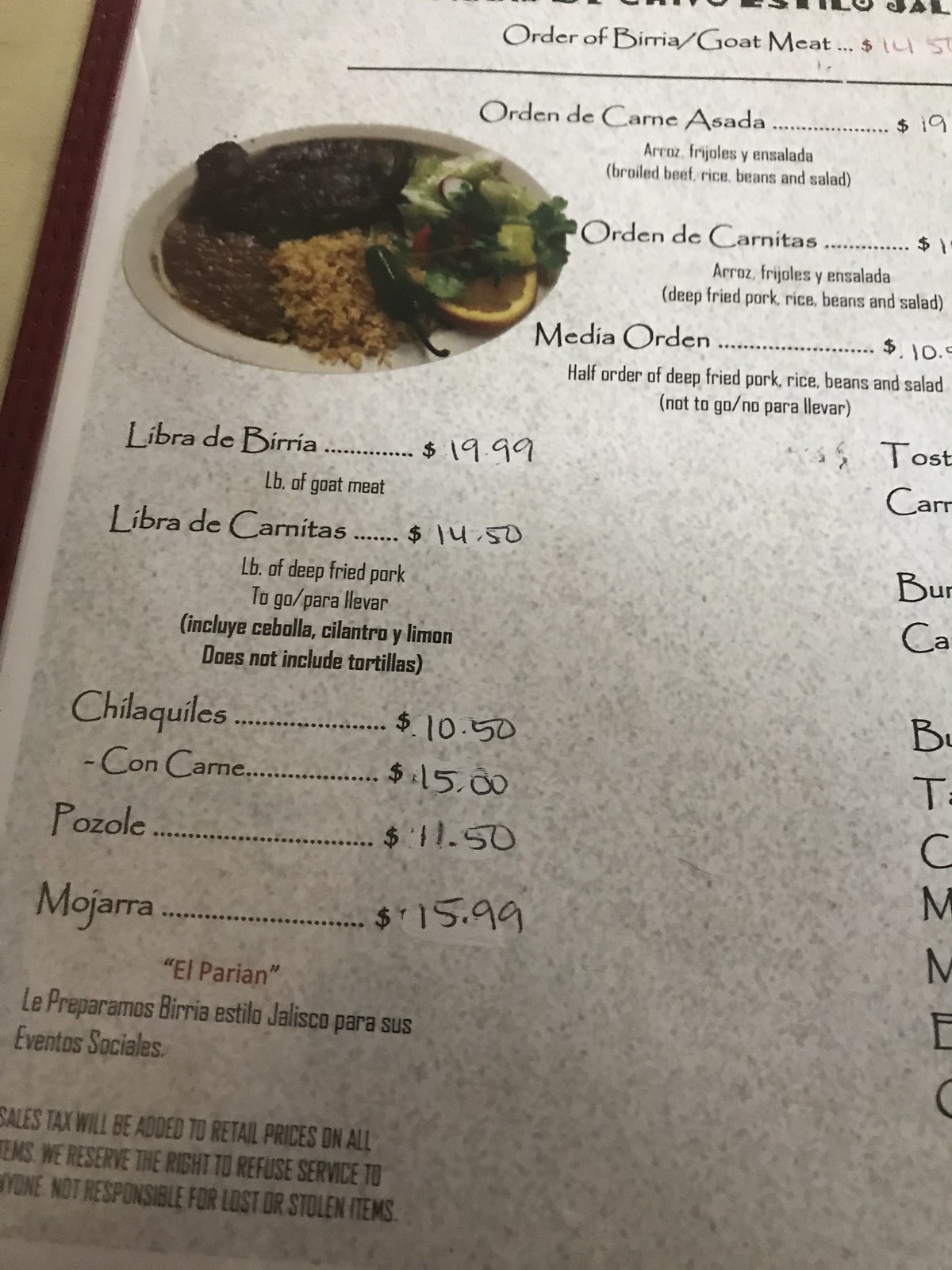The image depicts a portion of a menu placed on a tan surface. The top part of the menu isn't visible, so the name of the restaurant remains unknown. The menu features various food items along with their prices and descriptions, some of which are in Spanish.

At the top, there's an "Order of Birria/Goat Meat" priced at $14.50. Below it, there's "Orden de Carne Asada" for $19. This is followed by a detailed Spanish description. Next is "Orden de Carnitas," though its price is not visible. Underneath, a "Media Orden" (half order) priced at what looks like $10.50 is visible but partially cut off. It describes a half order of deep-fried pork served with rice, beans, and salad, with a note that it is not for takeout, accompanied by Spanish text. A plate pictured next to this section includes rice, beans, greens, citrus fruit, and dark-colored meat in the upper left-hand corner.

Further down on the left side, there is "Libra de Birria" priced at $19.99, translating to one pound of goat meat. The next item is "Libra de Carnitas" priced at $14.50, indicating one pound of deep-fried pork. Below this, more Spanish text appears. The menu continues with "Chilaquiles" priced at $10.50 and "Con Carne" at $15. Following this, "Pozole" is listed for $11.50 and "Mojarra" at $15.99. Below, "El Parian" is mentioned in Spanish, with a section discussing taxes at the very bottom.